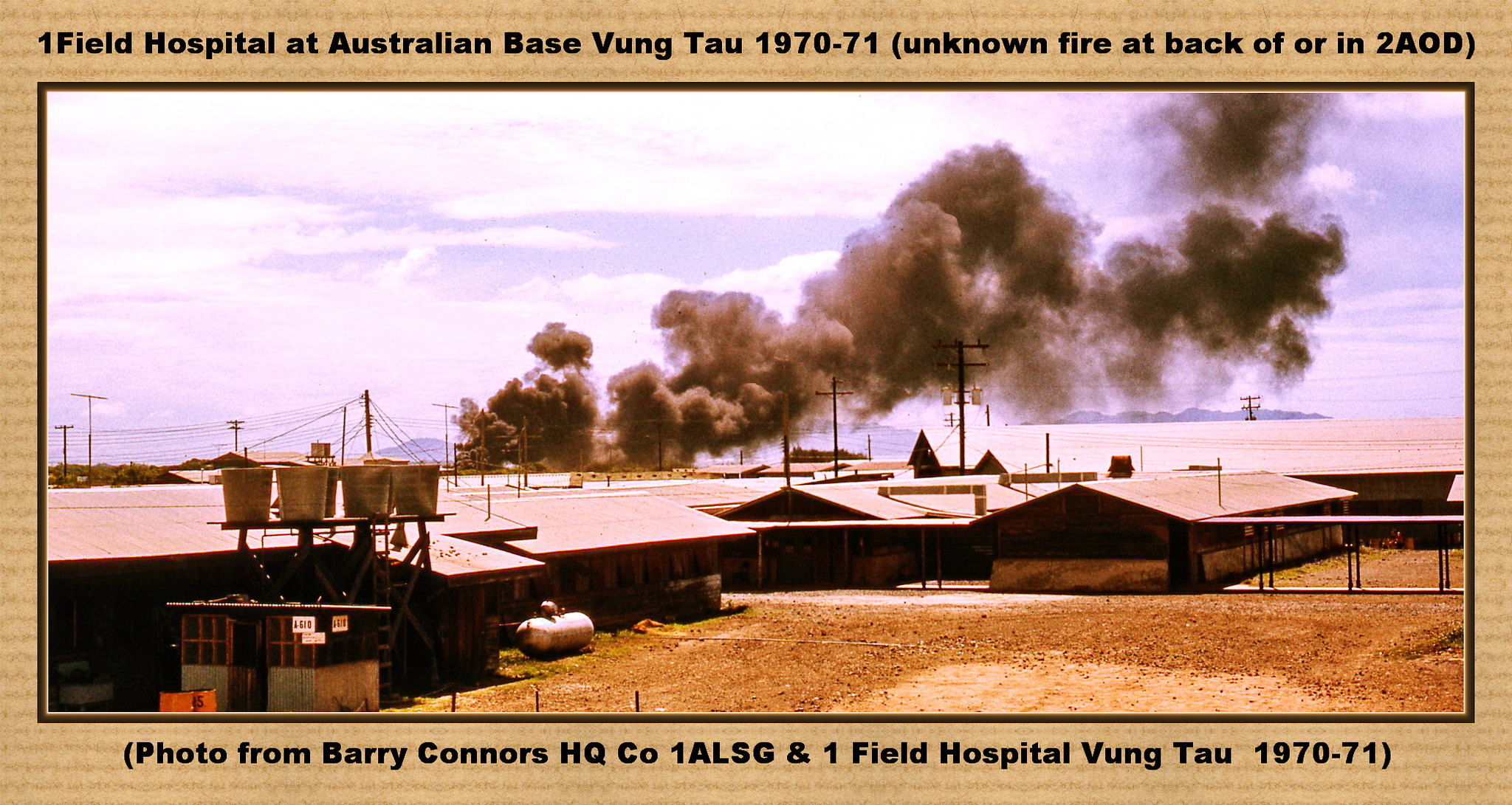This vintage photograph from 1970-71 depicts Onefield Hospital at the Australian base in Vung Tau, during an unknown fire incident. The image, credited to Barry Connors of HQCO 1ALSG, shows heavy, black smoke billowing from behind a series of closely packed, one-story buildings with metal roofs, suggesting a military hospital setup. In the foreground, a white tank with a red top—possibly for storing propane—sits outside one of the structures, amidst patches of brown grass and fenced-off areas. The scene captures a bare-bones, outpost style complex, interconnected with walkways and featuring power lines and transmitters. The backdrop includes hazy, cloudy skies and distant mountains. The image is bordered in black and set against a tan background with horizontal lines, highlighting its age and vintage quality.